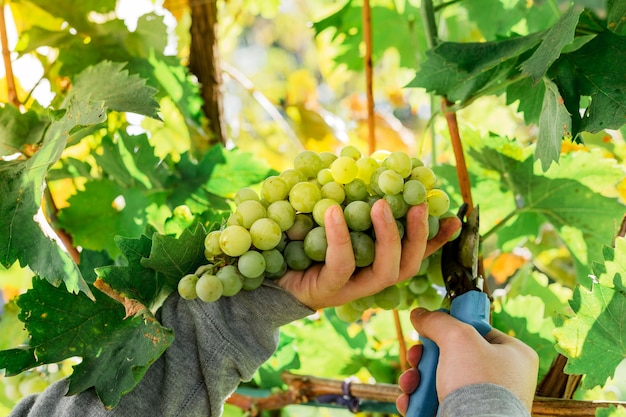This photograph captures a close-up scene of a Caucasian man harvesting ripe, green grapes in a vineyard. The man's left hand, clad in a gray long-sleeved sweatshirt, cradles a bountiful bunch of luscious green grapes that spill over the edges of his palm. His right hand, partially visible, holds a blue-handled pair of black cutting shears, skillfully snipping the grapes from a thin brown stem. The vibrant green leaves of the grapevine surround the cluster, accompanied by sunlit vines and additional grape foliage in the background, all bathed in a bright yellow glow. The scene is set outdoors, illuminated by sunlight, which highlights the natural beauty and ripeness of the grapes. The background features various grapevines and a small tree, adding depth and context to this vivid depiction of a fruitful harvest.